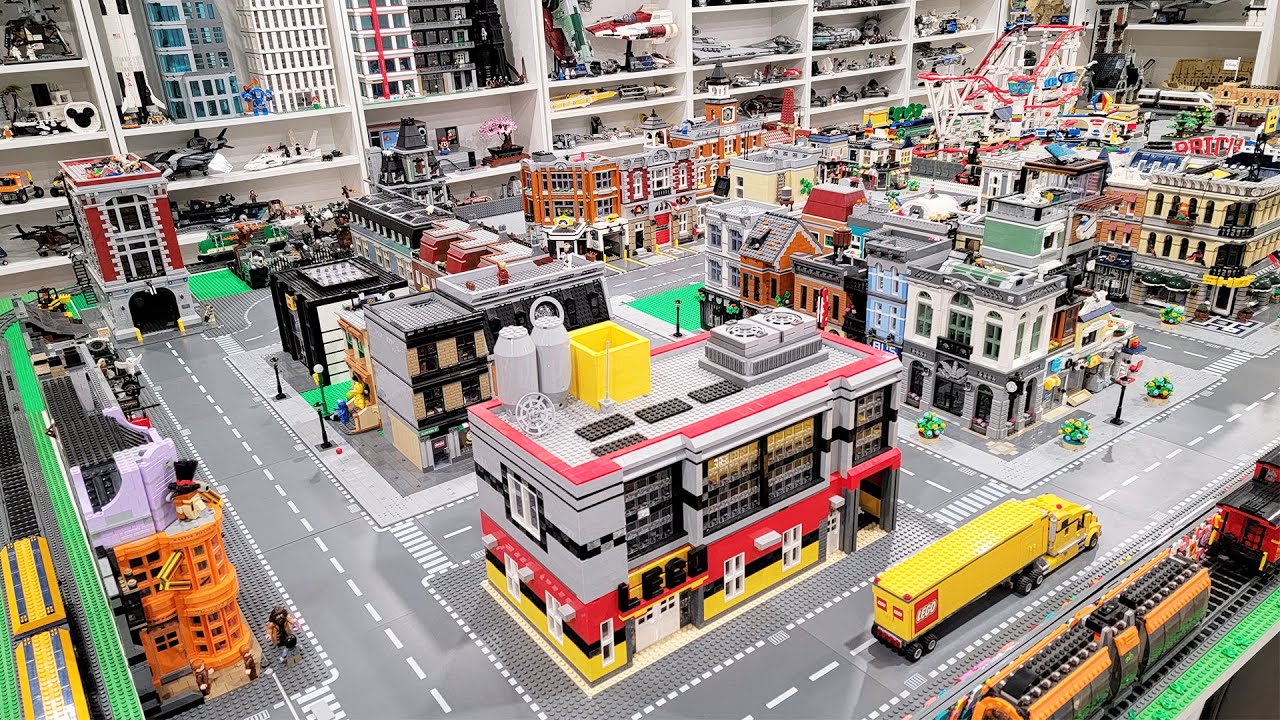The photograph depicts a detailed and impressive LEGO city setup, likely situated in either a hobby store or a dedicated room. The city features a vast array of buildings, including apartment complexes, storefronts, and townhouses, with meticulously paved roads threading through them. In the foreground, on a gray road, there is a prominent LEGO yellow tractor-trailer truck. Additionally, there is an eye-catching red and orange LEGO train visible in the bottom right corner. The upper right of the image showcases a cluster of brick buildings, adding to the urban landscape of the setup. Surrounding the LEGO city are white shelving units and cupboards filled with various toys and accessories, including Star Wars vehicles and other LEGO collectibles. The scene is vibrant with a multitude of colors, bringing the elaborate LEGO city to life.